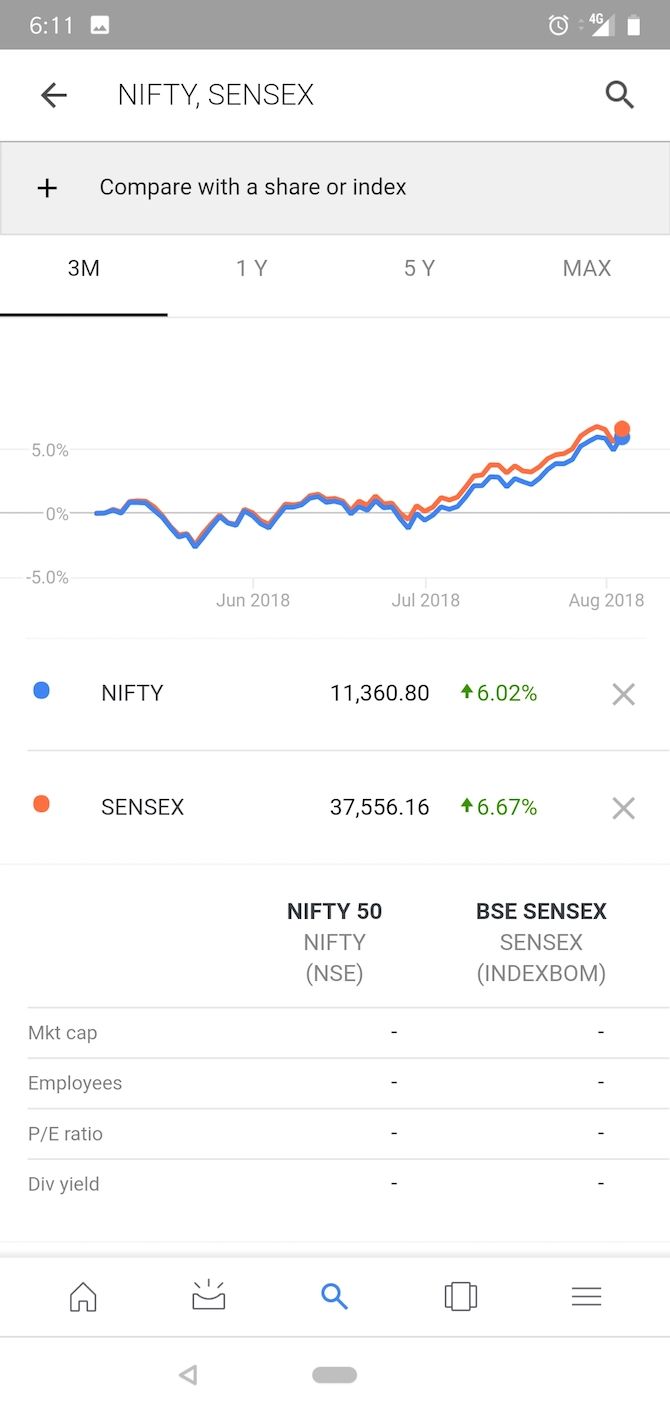Screenshot of a Stock Market App on a Smartphone

In the captured vertical portrait screenshot, the top section of the phone displays the status bar with several indicators: the time reads 6:11, a photograph icon, an alarm icon, a 4G network indicator that is about two-thirds full, and a nearly full battery meter. The main screen shows a stock market application with details about the Nifty and Sensex stock codes.

The user has selected to view stock performance over a three-month period. For the Nifty index, the current value is 11,360.80, which is up by 6.02%. The Sensex index is listed at 37,556.16, showing an increase of 6.67%. Below these indices, there are additional menu items: Nifty 50, Nifty NSE, BSC, Sensex, Sensex, and index bond.

Various financial metrics such as Market Cap, Employees, PE Ratio, and Dividend Yield are blank. The interface also includes navigation buttons for Home, Message, Search, and Minimize at the bottom of the screen.

The background of the app is plain white, with all text in black for clear visibility. A line chart depicting the growth of the stocks over the selected time period is prominently displayed, visually summarizing the upward trend.